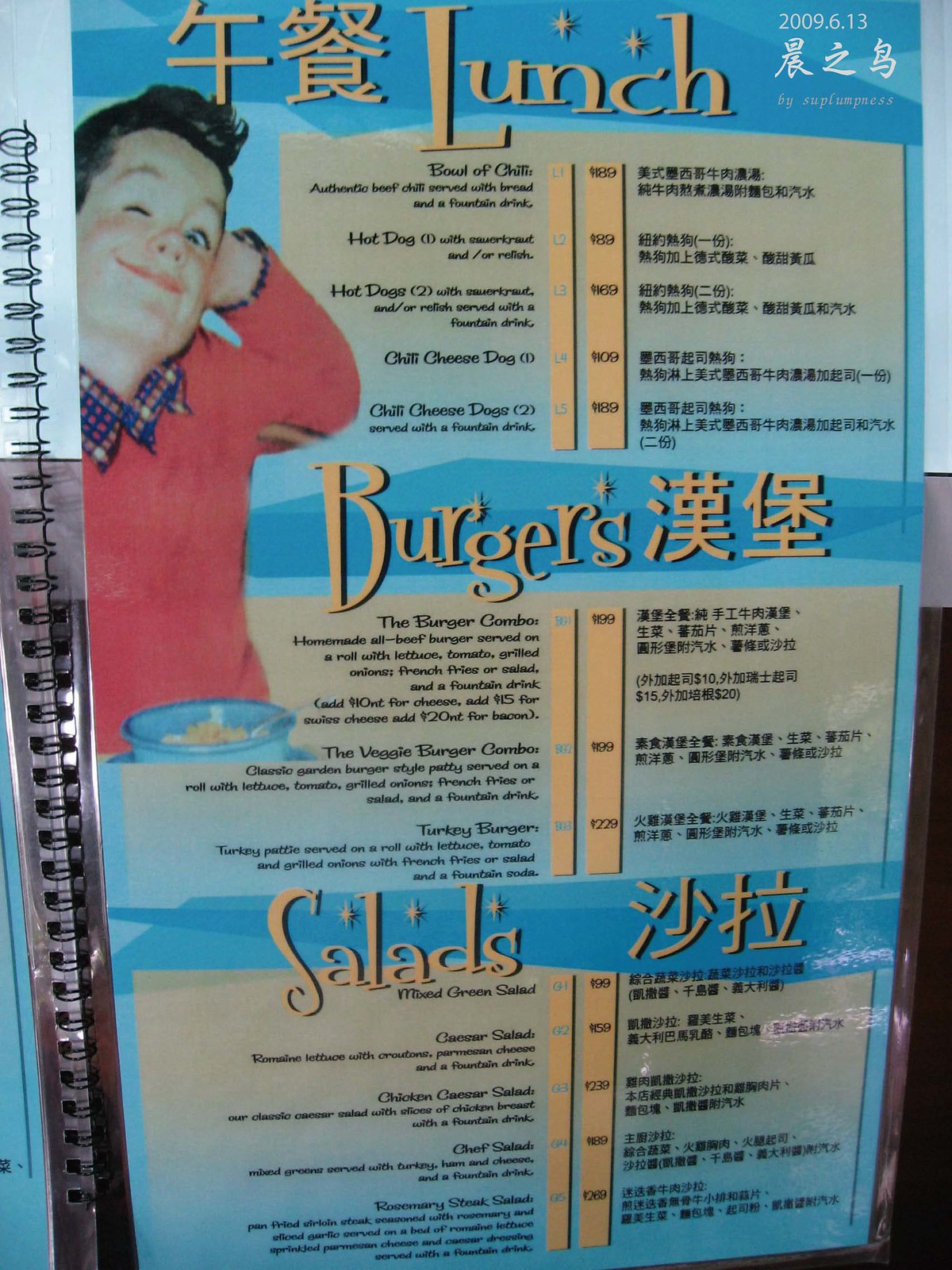The photograph captures a close-up of a menu page in portrait orientation, featuring a spiral binding along its left edge. The menu, written in both English and an Asian language, is set against a backdrop of varying shades of blue. Prominently, the upper left corner displays a photograph of a young boy. He is dressed in a red sweater layered over a blue, red, and yellow checked shirt, with the collar and an edge of the cuff visible. The boy, with dark hair styled back from his forehead, is leaning his head on his hand, smiling at the camera with one eye open and one eye closed. In front of him sits a blue bowl containing some brown food.

The menu is divided into three categories from top to bottom labeled as "Lunch," "Burgers," and "Salads," with category titles in a light orange font. Two vertical light orange stripes run down the center of the menu, seemingly indicating the prices. The left side of the page provides item descriptions in English, while the right side offers translations in an Asian language.